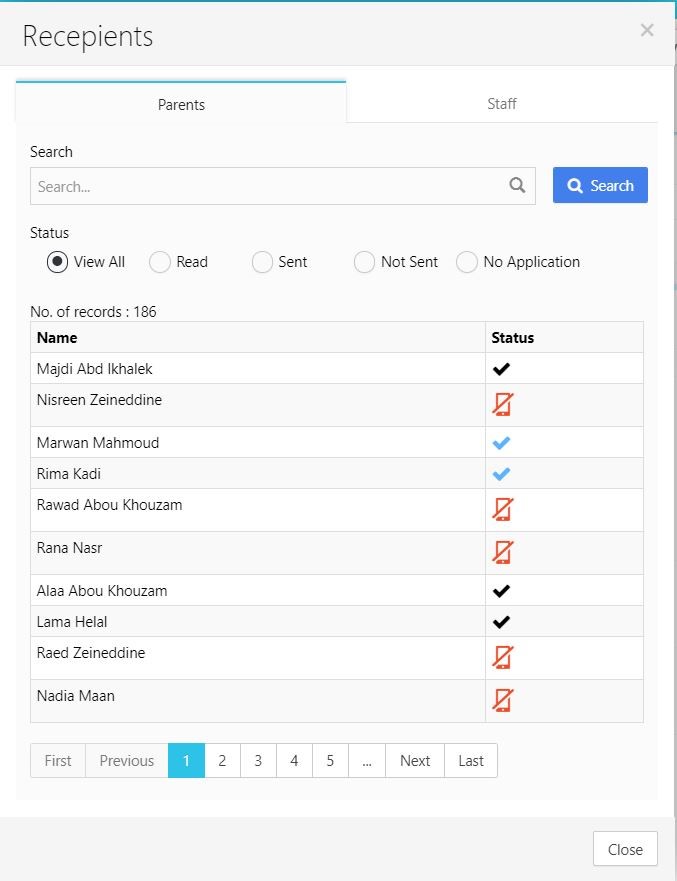On the webpage titled "Recipients," there is a typo – "recipient" is incorrectly spelled as "recepients." The correct spelling should be "recipients." The page features two main tabs: "Parents" and "Staff." Currently, the view is set to the "Parents" tab. Directly below, there's a search bar that allows for searching specific individuals. Presently, there are 186 records listed, and these are displayed over multiple pages.

The list predominantly features names that appear to be of Indian or Asian origin, such as Reema Khadi, Rana Nasir, and Lama Halal. Each entry is accompanied by a "Status" column on the right side. This column features various indicators, including black and blue check marks, as well as icons that resemble crossed-out phones. The check marks likely signify different types of statuses, while the crossed-out phone icon suggests that certain individuals may not have a phone number listed for communication. This system seems designed for managing parent contacts, likely for a school or educational institution.